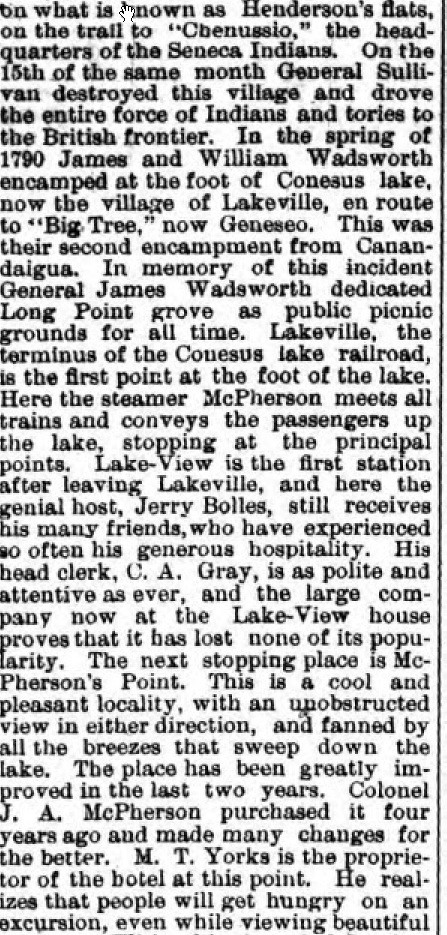The image depicts a single-column newspaper clipping displayed on a computer screen, featuring black text on a white background. The clipping recounts historical events and local history related to Henderson's Flats on the Trail to Chenusio—headquarters of the Seneca Indians. General Sullivan destroyed this village and forced the Indians and Tories to retreat to the British frontier on the 15th of an unspecified month. In the spring of 1790, James and William Wadsworth encamped at the foot of Canandaigua Lake, now the village of Lakeville, on their way to Big Tree, presently known as Geneseo. This marked their second encampment since they had left Canandaigua. To commemorate this event, General James Wadsworth designated Long Point Grove as public picnic grounds for perpetuity. 

Lakeville, the terminus of the Canandaigua Lake Railroad, serves as a central hub where the steamer MacPherson meets trains and ferries passengers along the lake, stopping at major points. The first stop is Lakeview, where the hospitable Jerry Bowles and his polite head clerk, C.A. Gray, welcome guests at the Lakeview House. The next stop is MacPherson's Point, which boasts clear views in all directions and has been significantly improved over the past two years under the ownership of Colonel J.A. MacPherson. The hotel at this location, managed by M.T. Yorks, caters to the needs of travelers who want to dine while enjoying the picturesque scenery.